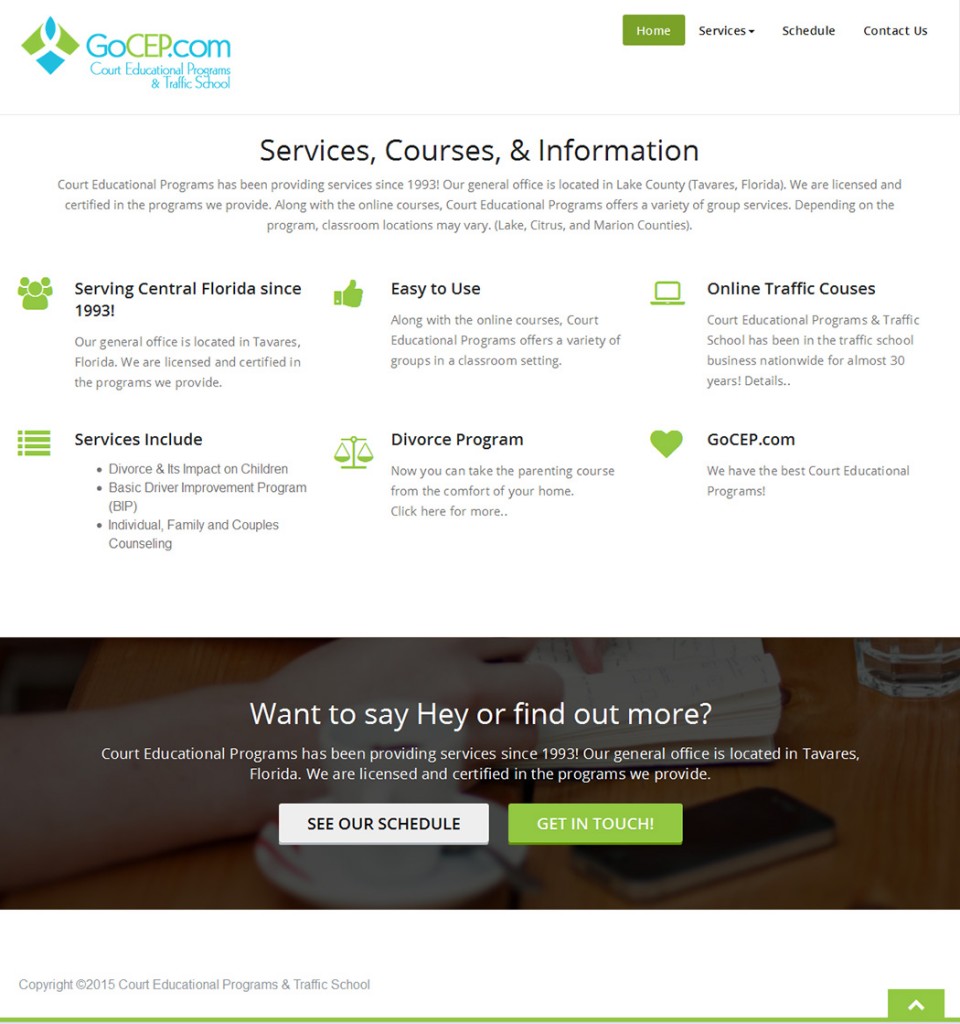In the upper right-hand corner of the website, there is a turquoise text displaying the URL "GoCEP.com" with "CEP" in green, all capital letters. To the left of the web address, there is a logo in turquoise and green. Located just below the web URL, the site reads "Court Educational Programs and [distorted text]" with the rest being unreadable.

On the right side of the page, there is a navigation menu featuring clickable options: "Home," "Services," "Schedule," and "Contact Us." The "Services" tab has a small down arrow next to it, indicating a dropdown menu. The "Home" button stands out with white font against a green rectangle background, while the remaining options are in black font.

Centrally positioned on the page, bolded black text titles the section: "Services, Courses, and Information." Below, a paragraph reads: "Court Educational Programs has been providing services since 1993. Our general office is located in Lake County (Tavares, Florida). We are licensed and certified in the programs we provide. Along with online courses, Court Educational Programs offers a variety of group services. Depending on the program, classroom locations may vary (Lake, Citrus, and Marion Counties).”

Beneath this, six items are presented in two horizontal lines, each accompanied by a green icon to the left of the heading:

1. "**Serving Central Florida since 1993**"
   - "Our general office is located in Tavares, Florida. We are licensed and certified in the programs we provide."
   
2. "**Easy to use**"
   - "Along with the online courses, Court Educational Programs offers a variety of groups in a classroom setting."
   
3. "**Online traffic courses**"
   - "Court Educational Programs and traffic school has been in the traffic school business nationwide for almost 30 years. Details."

The second line highlights:

4. "**Services include**"
   - Bullet points:
     - "Divorce and its impact on children"
     - "Basic Driver Improvement Program (BIP)"
     - "Individual, family, and couples counseling"
   
5. "**Divorce program**"
   - "Now you can take the parenting course from the comfort of your home. Click here for more."

6. "**GoCEP.com**"
   - "We have the best court educational programs," with a green heart icon next to "GoCEP.com."

At the bottom of the website, a horizontal rectangular area displays white font reading: "Want to say hey or find out more?" This is followed by further details, and two horizontal rectangles with call-to-action buttons: a white button with black font stating "See our schedule," and a green button with white font reading "Get in touch."